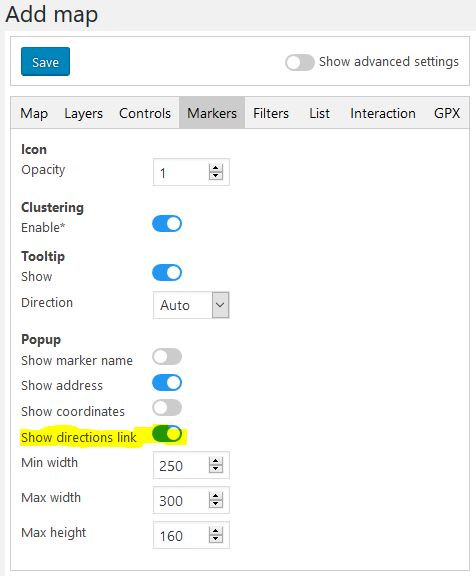This screenshot captures the settings interface of an application. At the top, there's a light gray bar with large black font on the upper left stating "Add Map." Directly below, a white rectangular section is displayed. 

On the left side of this section is a purple rectangle labeled "Save" in white font. To the right, there's a toggle switch labeled "Show Advanced Settings." 

Beneath this, there's another gray rectangle containing several options: "Map," "Layers," "Controls," "Markers," "Filters," "List," "Interaction," and "GPX." The "Markers" option is selected and highlighted in a darker gray.

Within the "Markers" settings, various configurable options are displayed. These include:
- "Icon Opacity" with a drop-down menu where a selection has been made.
- "Clustering" option, which is enabled.
- "Tooltip" option, also enabled, showing "Show Direction" with an "Auto" drop-down menu.
- A "Pop-up" section with several toggles:
  - "Show Marker Name" is toggled off.
  - "Show Address" is toggled on.
  - "Show Coordinates" is toggled off.
  - "Show Directions Link" highlighted in yellow and toggled on.

At the bottom, there's a section for dimensions, showing "Max Width" and "Max Height" settings, specified as 250, 300, and 160 respectively.